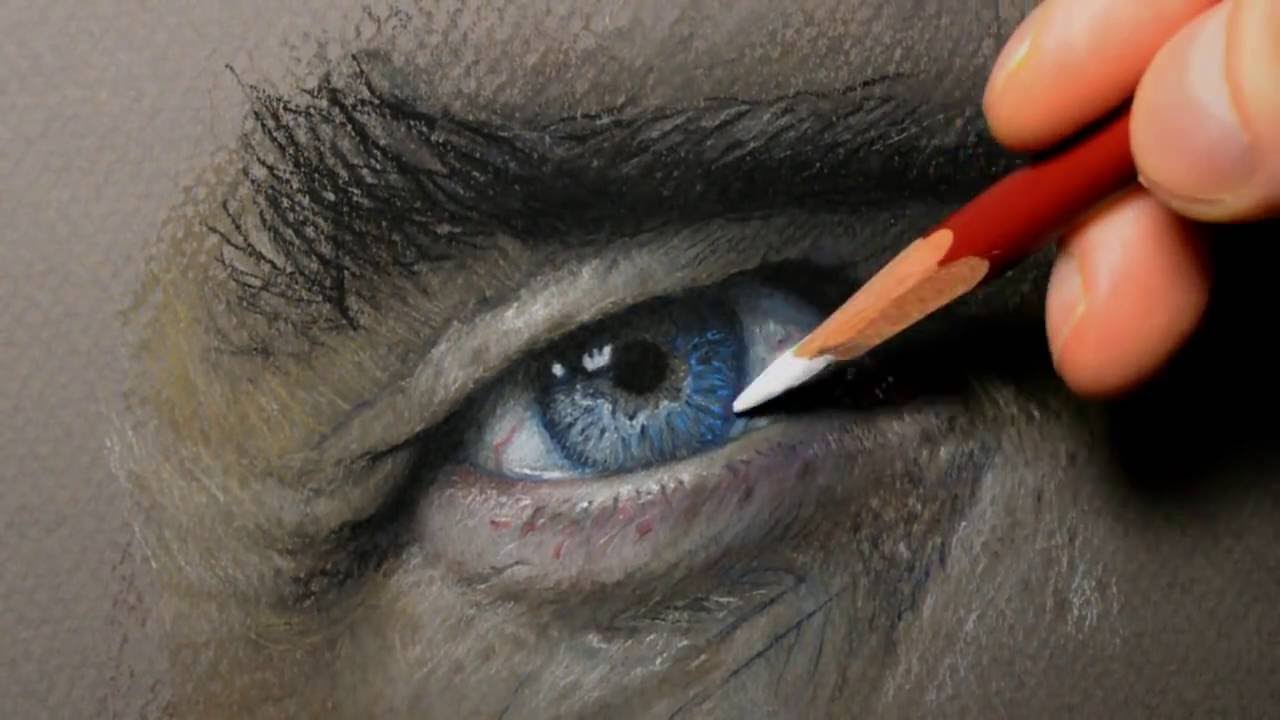The photograph captures a highly detailed close-up of an artwork depicting a human eye, seemingly drawn with colored pencils on a textured canvas. At the center of the composition is a blue eye with a black pupil, surrounded by the whites of the eye. The eye appears hooded and is framed by dark, bushy eyebrows at the top and sparse, delicate eyelashes at the bottom. The edges of the image reveal an unfinished texture indicative of an ongoing art project.

In the top right corner of the photograph, a hand is poised, holding a red colored pencil with a white tip. Only three fingers are visible, applying the white pencil directly to the whites of the eye in the artwork. The background of the image is a tannish skin tone, further emphasizing the central focus on the intricate details of the eye being meticulously colored and shaded. The absence of any textual elements or writing within the photograph suggests that the scene is purely about the artistic process of drawing and detailing the human eye.